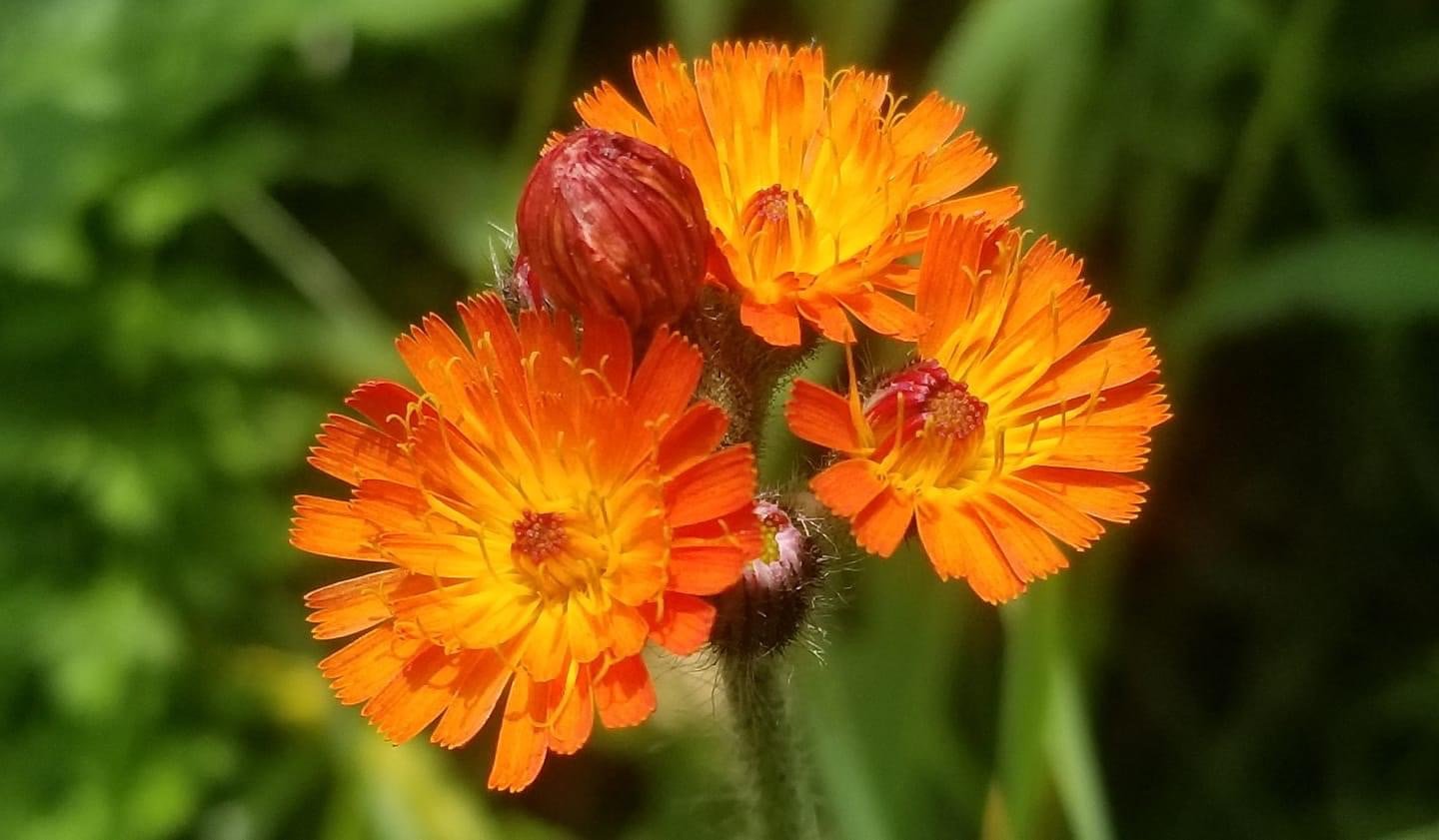This captivating photograph, likely the work of a skilled wildlife or nature photographer, features three vibrant flowers in full bloom with a fourth bud yet to open. The flowers showcase striking orange petals that transition to a lighter yellow towards their amber-orange centers. One of the stems hosts a black insect with a white head and a hint of red. The background offers a verdant display of green foliage, bathed in sunlight with occasional areas of shadow. The greenery, which includes trees, plants, and bushes, appears somewhat blurred, creating a soft, natural backdrop. On the right side of the image, a dark background provides contrast, enhancing the vivid colors of the flowers and the sunlight illuminating them. The intricate details and interplay of light and shadow bring a serene and enchanting quality to the composition.